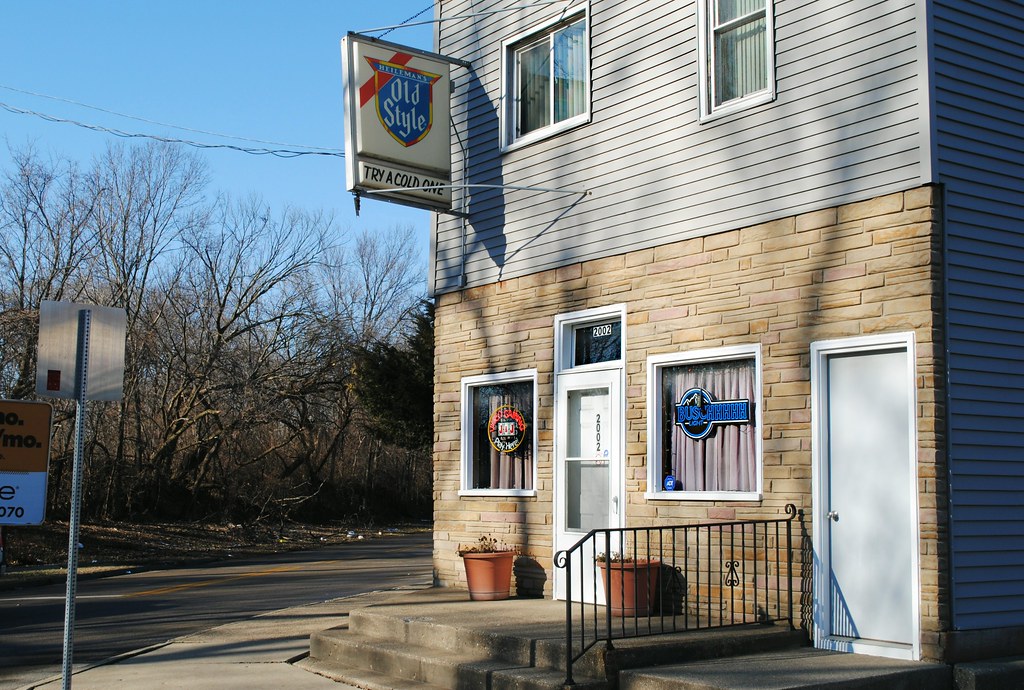This photograph captures a small tavern located in a suburban or rural town. The tavern, featuring a utilitarian design, occupies a building with a distinct two-tone exterior: the lower walls are brown, while the upper portion is clad in gray siding. The facade boasts a classic charm, with white concrete steps leading up to the main entrance. Flanking this door are two windows, each showcasing neon signs from various beer makers, including a prominent red-on-yellow circular sign on the left and a blue "Bush Light" sign with an extended "H" on the right. A small window above the door displays the building number, 2002.

To the right of the main entrance, another window is partially obscured by a metal railing, suggesting a possible secondary entrance. This side door appears to lead to an upper floor, reinforcing the building's multi-use potential. Plant pots in red hues decorate the exterior, adding a splash of color. Meanwhile, on the left side of the photo, a road stretches away from the viewer, adorned with a few signboards and flanked by leafless trees, all under a clear blue sky. Above the tavern’s door hangs a sign that reads "Heilman's Old Style," inviting passersby to "Try a Cold One," thus enhancing the building’s welcoming yet straightforward appeal.